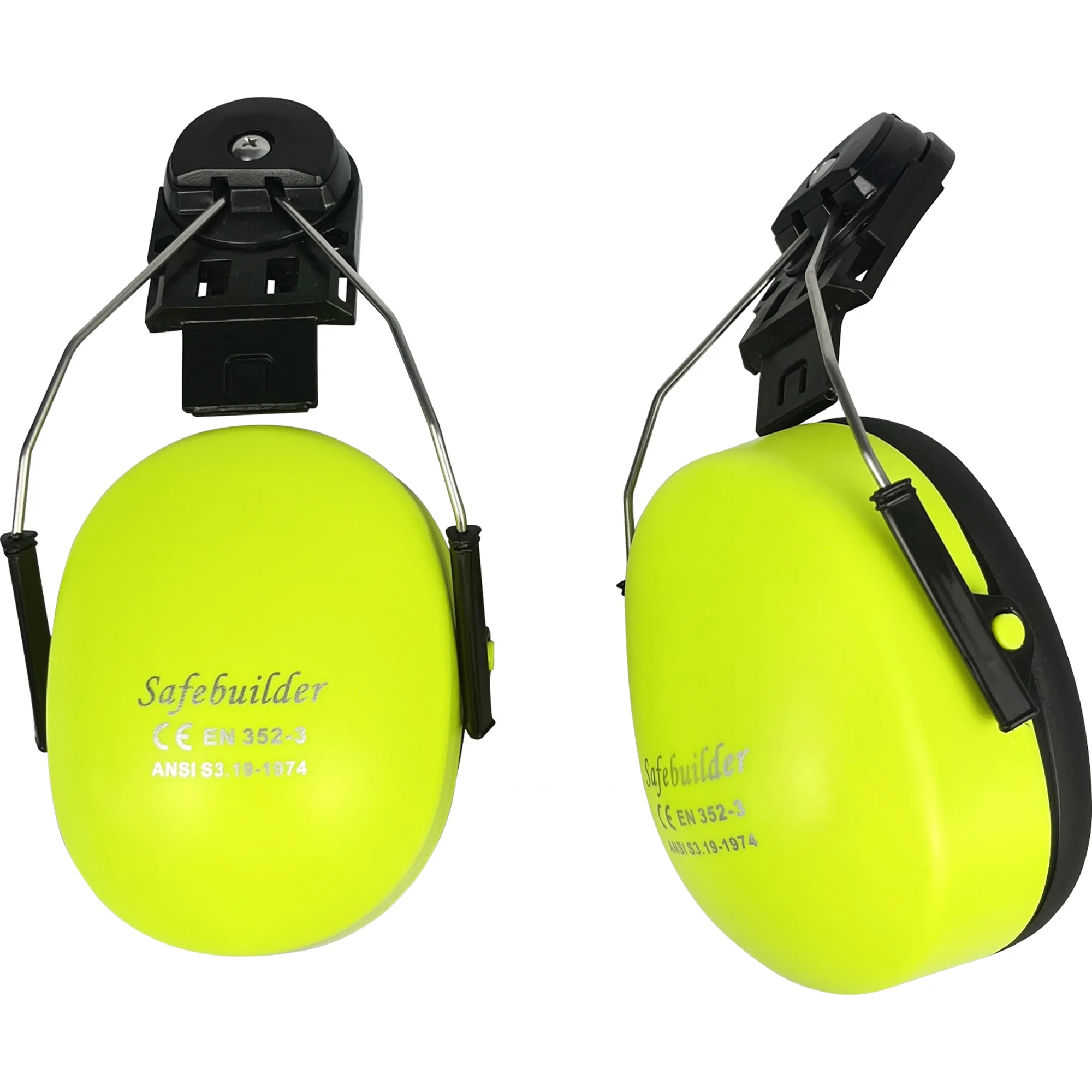This image shows two photographs of safety headphones, displaying both a front and a side view of the ear cuffs against a plain white background. The headphones, which are a bright lime-yellow, have black and silver wires attached at the top, secured by screws. The top part where the headband would attach is black. The text on the ear cuffs reads "SafeBuilder," followed by "CEN352-3," and beneath that, "ANSI S3" with additional numbers that are partially obscured due to glare, making them difficult to read but include "1974." The image highlights the details of the headphones' structure, including the dual metal and plastic components that connect to metal rods extending upwards where the headband would be.